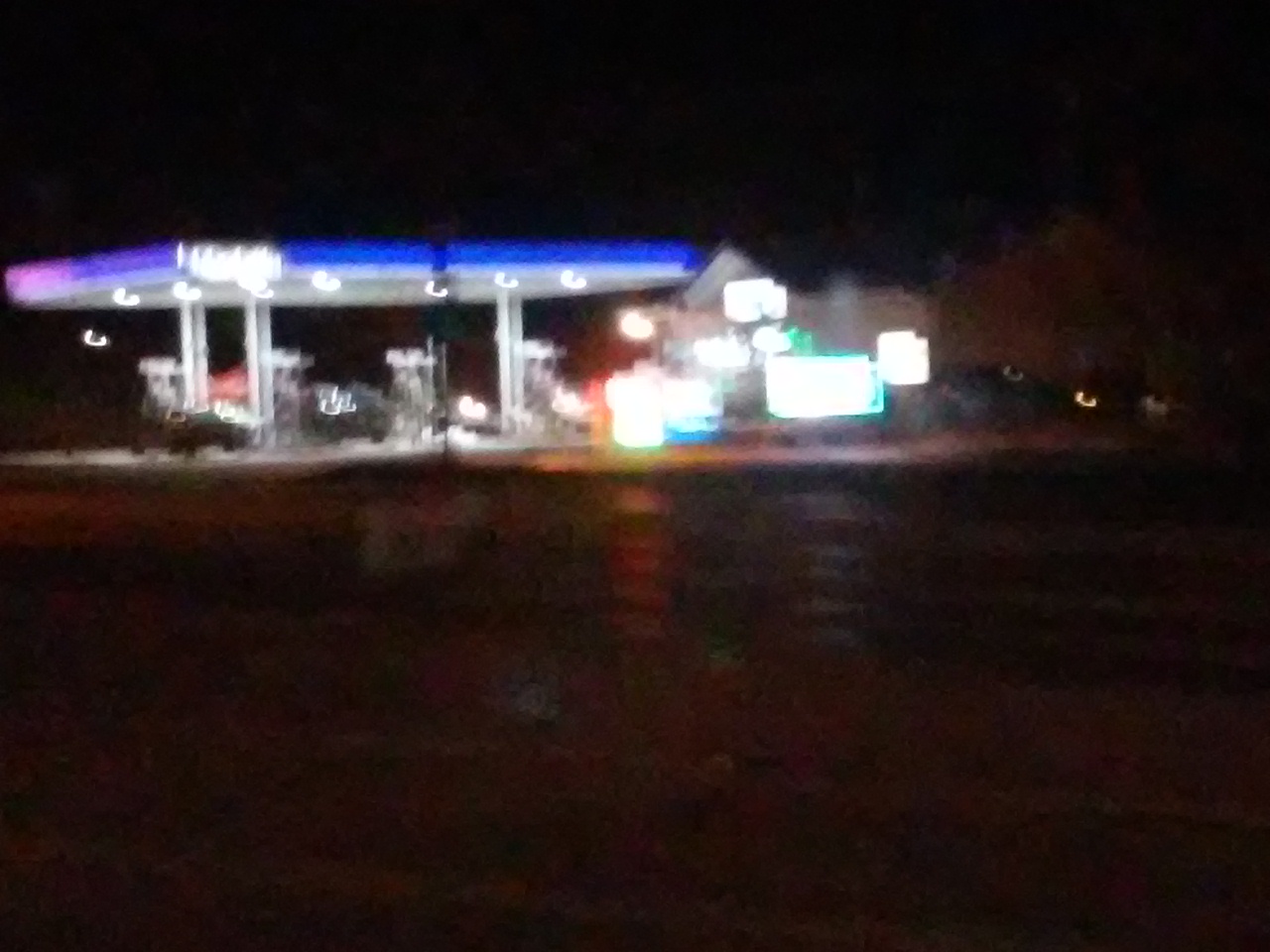The image captures a nighttime scene at a gas station and possible convenience store, with a bit of rain suggested. The surroundings are blurry and grainy, likely due to motion and light reflections. The foreground is dominated by a road leading into the gas station, which features a large canopy with distinctive blue and, possibly, pinkish-purple lights at the top, illuminating the gas pumps and a few indistinct cars refueling underneath. To the right, a larger structure which might be a grocery store rather than a simple convenience store extends, marked by white or gray walls and various signs and lights. The bright lights from both the canopy and the building create a glowing effect, adding to the haze and making details difficult to discern. Cars are present both at the pumps and around the building, contributing to the bustling yet fuzzy night-time atmosphere.